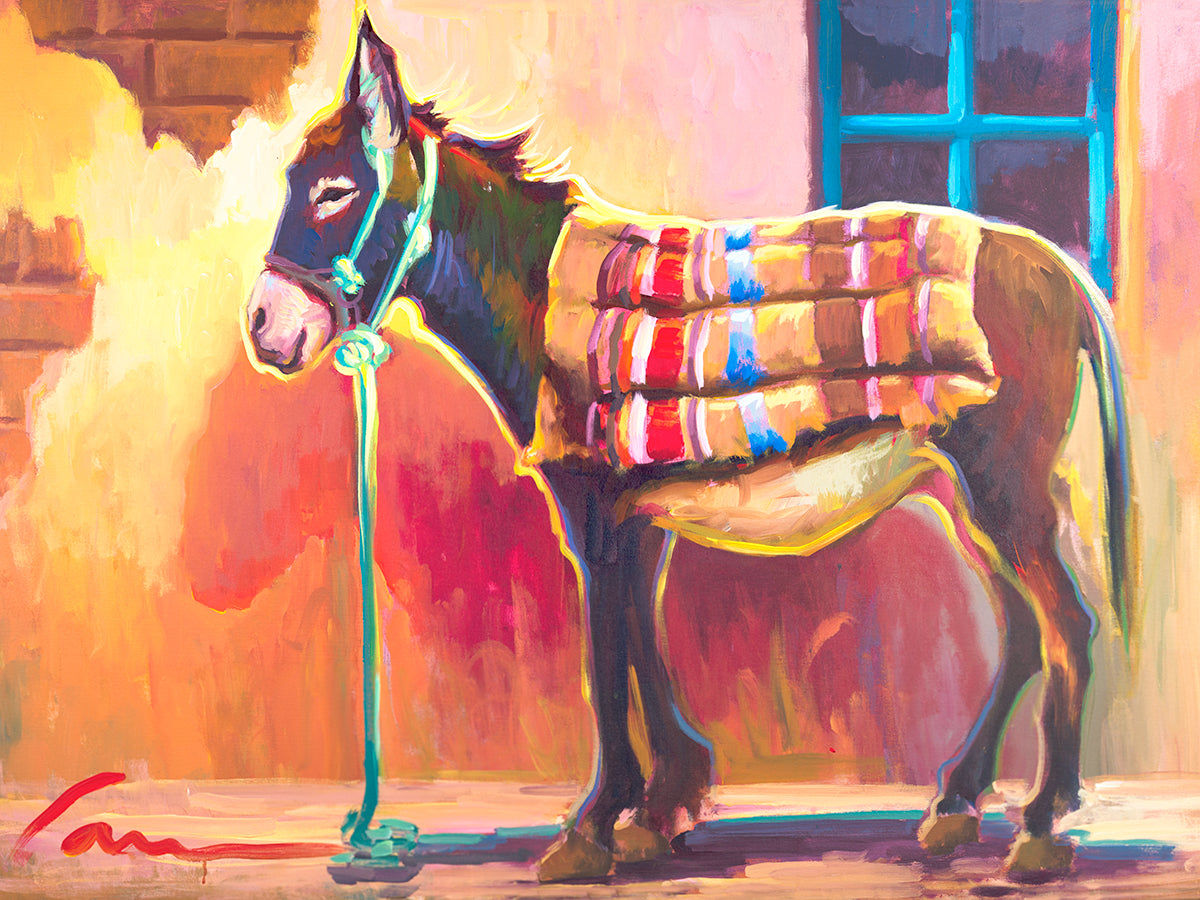This is an intricately detailed oil painting of a brown donkey standing in profile, looking to the left. Draped over its back is a multi-colored poncho-like blanket with prominent stripes of beige, rust, white, red, purple, and blue. The donkey is adorned with a green harness and a matching leash that hangs down to the floor. The scene is set against an adobe-style structure that features a mix of exposed bricks and softer, lighter wall colors that contrast starkly with the vibrant blue painted window. The artist’s signature, marked in red, is located at the bottom left of the painting. The overall use of hot and cold colors creates a striking visual effect, enhancing the Spanish or Mexican-inspired aesthetic of the artwork. The donkey, with its protruding belly and short mane, stands contentedly, adding to the quaint and cheerful atmosphere of the scene.